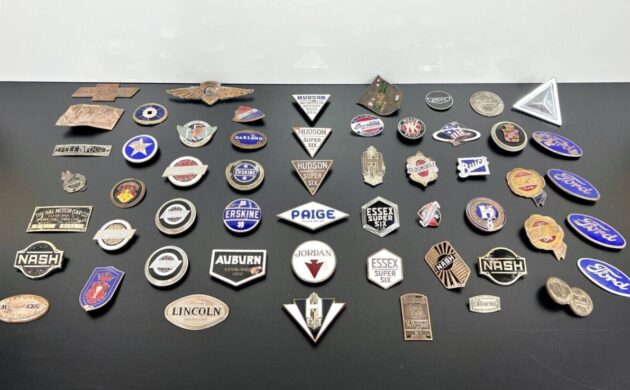The image depicts a vintage collection of approximately 30 pin buttons and stickers, meticulously laid out on a dark, predominantly black tabletop with hints of gray. These pins are an eclectic mix of shapes and colors, many showcasing automotive brands. Notably, there are multiple Ford logo pins—at least four—while other recognizable names include Nash, Lincoln, Page, Essex Super 6, Jordan, and Auburn. Among the diverse shapes are circles, stars, shields, and various ones with wings; some pins are in good condition while others show signs of rust and wear. The color palette is quite muted, dominated by beige, black, white, and some blue. While some pins feature text like Hudson, Erskine, Audubon, and Buick, a round pin with the Nash logo stands out prominently. There is also a barely visible pin in the background that might represent the New York Yankees. Overall, this vintage assortment gives a nostalgic nod to early car memorabilia.